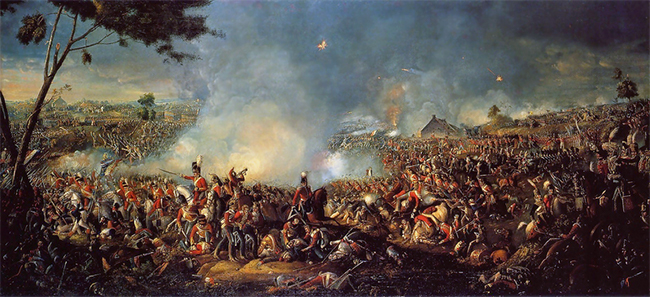The rectangular horizontally oriented painting depicts a chaotic Revolutionary War battle scene. The background is dominated by a smoky, gray sky interspersed with orange and yellow fire spots, possibly from explosions. To the far left, green foliage and a tree branch with pine needles add a touch of nature. Farmhouses and a barn are visible in the distance amidst the smoky landscape. 

In the foreground, hundreds of British redcoats in red and white uniforms with distinctive black hats and feather plumes are seen in action. Soldiers on horseback, some brandishing swords and directing troops, intermingle with those running with guns and tending to the wounded. Many lie on the ground, either injured or dead. The image also captures a moment of intense battle, with dark clouds of smoke rising from the apparent blasts on the ground.